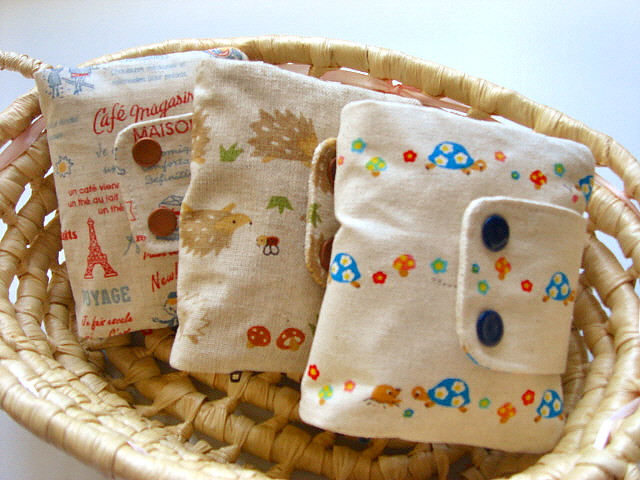The image features a simple, small, oval wicker basket with a light, woven appearance, set against a white background. Inside the basket are three hand-sewn pouches, each with a distinct design and clasped with snap buttons. The pouch on the left prominently displays the text "Café Maison" in red letters, alongside various French-themed images, including the Eiffel Tower. The central pouch showcases a nature-inspired design with brown porcupines, red-tipped mushrooms, and possibly bees or ladybugs. The right-hand pouch is adorned with blue-shelled turtles decorated with white flowers and multicolored mushrooms, including red and green ones. Each pouch features a flap that snaps shut, adding a functional yet decorative touch to their charming and detailed patterns.